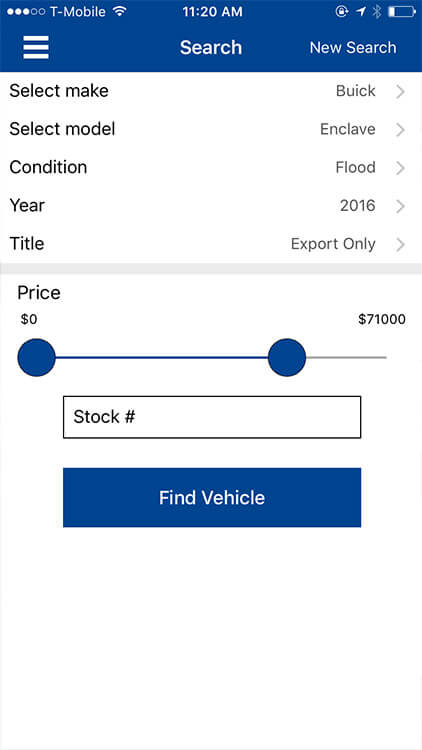Screenshot of a mobile device screen taken vertically and displaying an automotive search interface. 

- At the top, a blue status bar shows the time as 11:20 AM. On the left side of the bar, "T-Mobile" with a 3 out of 5 signal strength indicator is visible. On the right side, the battery icon indicates approximately 20% charge.
- Directly below the status bar, there is a search bar with an icon on the right.
- Beneath the search bar, the text fields display:
  - "Make" with "Buick" selected,
  - "Model" with "Enclave",
  - "Condition" tagged as "Flood",
  - "Year" set to "2016",
  - "Title" noted as "Export Only".
  Each field has a small gray arrow pointing to the right, indicating they are selectable for more options.
- Below these options, a thin horizontal gray bar separates the filters from the pricing section.
- The "Price" section is a slider labeled from $0 on the left to $71,000 on the right, with two blue circles marking the selection range. One circle is at $0, and the other is approximately two-thirds along the bar, connected by a blue line.
- Under the price slider, there is an input box labeled "Stock Number".
- At the bottom, a prominent blue button with white text reads, "Find Vehicle".

This descriptive caption provides comprehensive details of the mobile interface for vehicle search, including the status bar, filter options, and interactive elements.